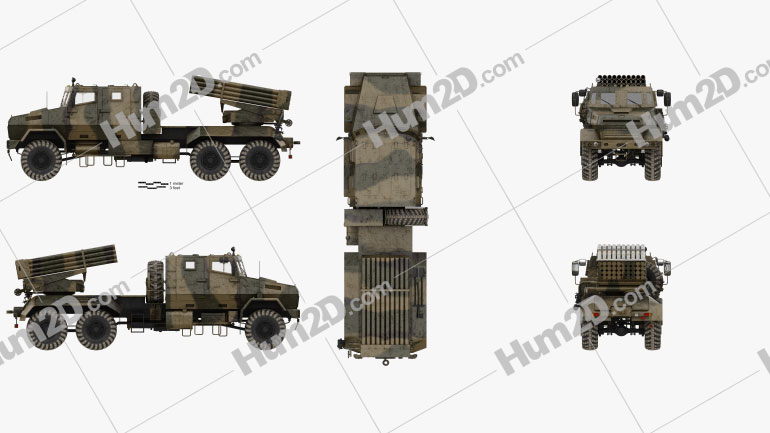The image showcases a military truck from five different angles against a background of solid light gray with diagonal lines and the text "HUM2D.com" repeated throughout. The military truck, depicted in both a darker dull green and a lighter dull green camouflage pattern, features large tires—three on each side—totaling six, including a spare tire. The vehicle has a slightly raised back bed which appears to be equipped with a missile or cannon-like structure. The views are organized as follows: the side view on the upper left, an opposing side view below it, a top view in the center, the front view in the upper right corner, and the back view in the bottom right corner. The image is overlaid with a transparent grid, reinforcing the military and technical aesthetic of the depiction.